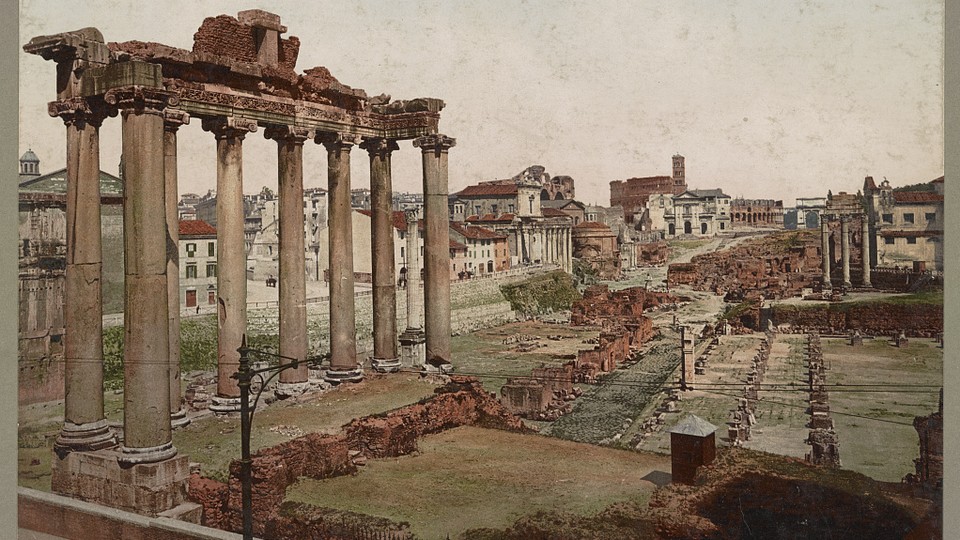This image, which appears to be either a very old photograph or an artist's illustration, showcases an excavation site reminiscent of ancient Rome, possibly the Roman Forum. The scene is dominated on the left by eight tall, ornate Grecian columns, likely remnants of a significant building such as the Temple of Jupiter. These columns support fragments of a crumbling roof, with much of the structure having fallen away, leaving only parts of the foundation visible. To the right of these columns are shorter brown brick walls and additional ruins scattered across a small open field. Beyond this field stands another set of columns and further remnants, emphasizing the site's historical decay.

In the background, a collection of graying white and red-roofed modern buildings stretches towards the horizon, blending into a grayish-white sky. A few power lines and an old-fashioned telephone pole suggest some dated infrastructure, indicating the photograph or illustration could be from the early 20th century. The entire scene is streaked with age, featuring gray splotches that add to its antiquated appearance. The coloration in the image includes various shades of brown, green, and brick red, lending a realistic, if weathered, depiction of the ruins and their juxtaposition against the encroaching modern town.